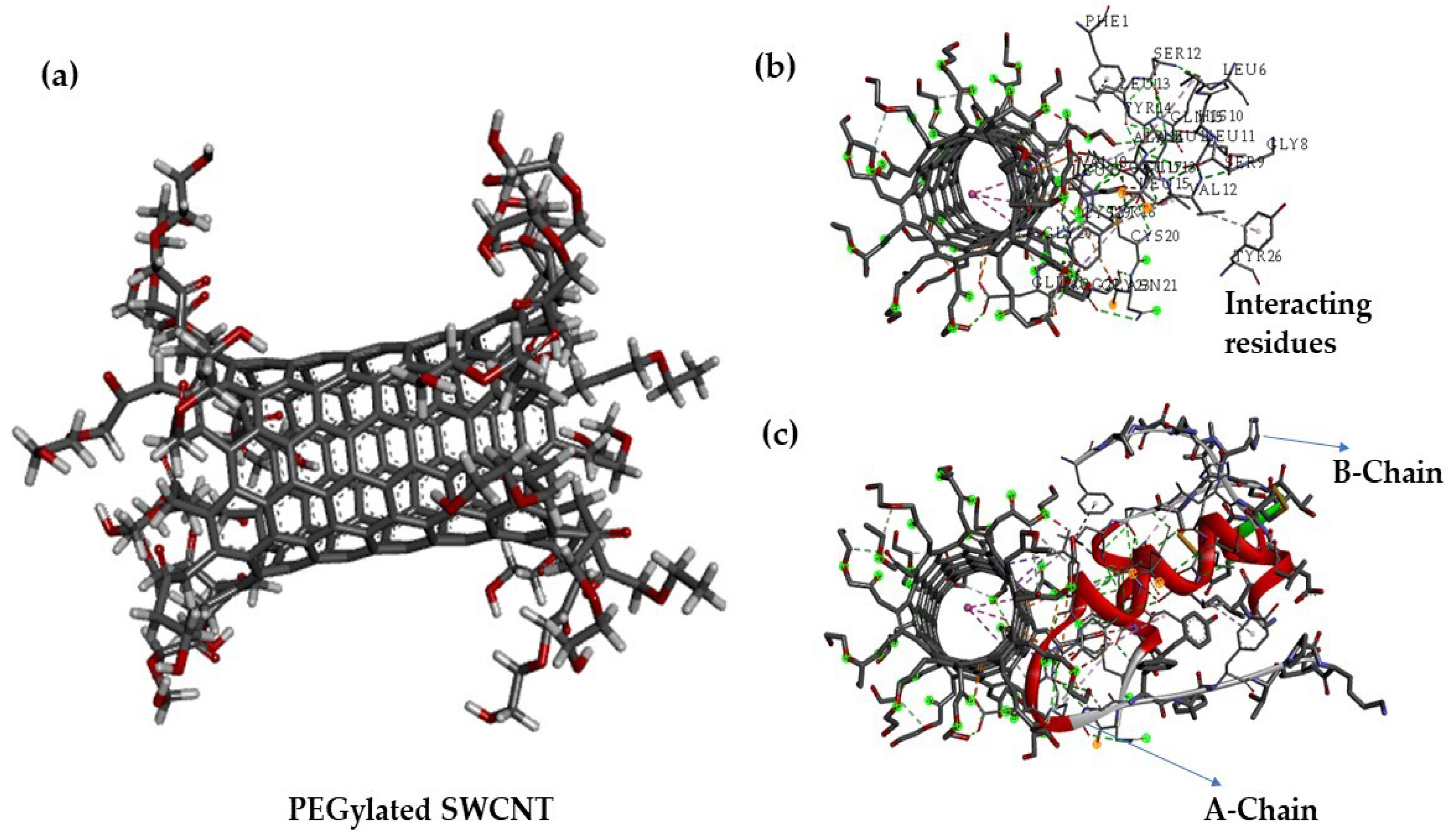This image showcases three distinct stations labeled A, B, and C. 

Station A features a configuration of small wire clips assembled into a rectangular shape, with additional protrusions extending from each of the four corners. This station is labeled "PEGylated SWCNT," indicating the use of polyethylene glycol-functionalized single-walled carbon nanotubes.

Station B illustrates a circular wire structure from which multiple individual wires emanate in all directions. This setup is designated as "Interacting Residues," hinting at a molecular interaction or binding site analysis.

Station C presents two chains, labeled "A chain" and "B chain," with a prominent red channel running through the structure. This is associated with a circular element with extending pieces, possibly representing a complex molecular or protein interaction.

The detailed imagery in all three stations highlights different molecular configurations and interactions, contributing to a comprehensive understanding of the depicted scientific phenomena.